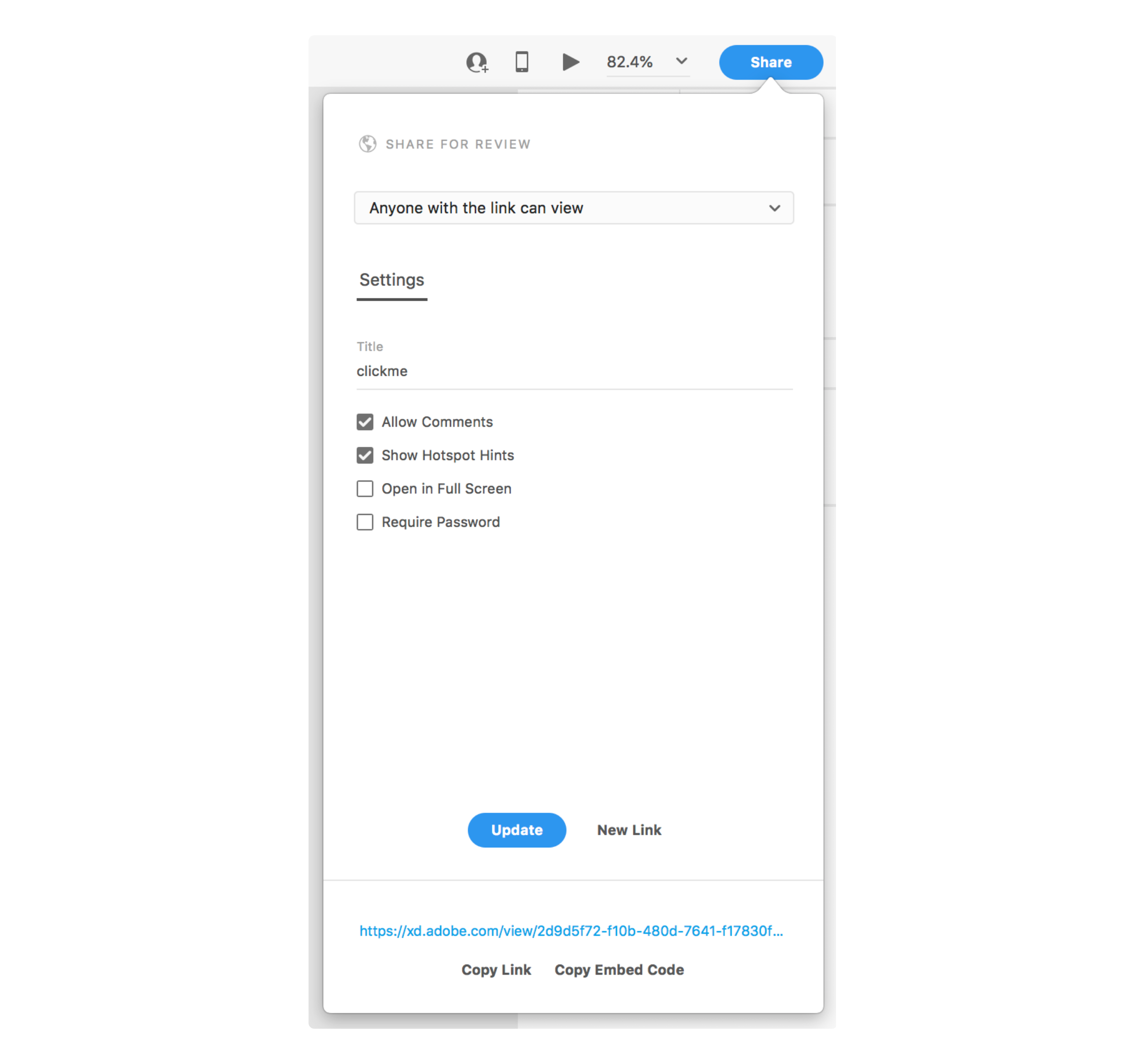This image depicts a vertically oriented mobile screenshot showcasing a white pop-up box with various features and options for sharing content. At the top of the image, there's a very light gray navigation bar featuring a profile icon, a phone icon, and a gray right arrow icon. Additionally, there's a scroll bar indicating 82.4% and a blue "Share" button.

Below the navigation bar is a large white pop-up box. At the top left corner of this box, it reads "Share for review" accompanied by a globe icon. Below this, a horizontal scroll-down bar indicates the setting "Anyone with the link can view." Directly beneath this bar, on the left, is an underlined "Settings" label.

A space for the title follows, with "ClickMe" entered as one word. Proceeding downward, there are four checkboxes, with the first two boxes—"Allow comments" and "Show hotspot hints"—checked. The next options available for selection are "Open in full screen" and "Require password."

At the bottom-center of the pop-up box is a small blue "Update" button next to the text "New link." To the box's extreme bottom, there is a long blue text link leading to adobe.com, followed by options "Copy link" and "Copy embed code."